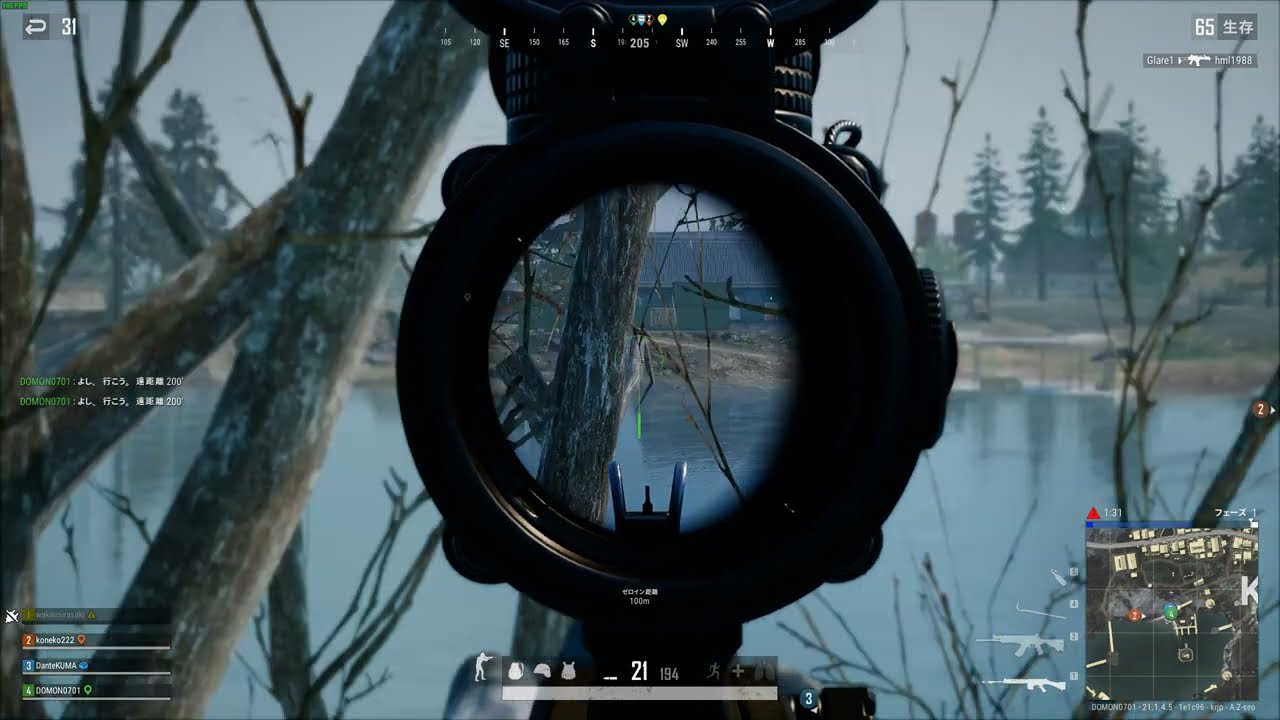This image captures a detailed screenshot from a first-person shooter video game, viewed through the scope of what appears to be a sniper rifle. In the center of the screen, the crosshairs of the scope focus on a distant building, partially obscured by foreground branches, suggesting the sniper is taking cover behind some trees. Below, various HUD elements are visible: ammunition count, life, and energy indicators span the bottom, while a mini-map of the area, populated with user icons and marked in shades of green and orange, occupies the bottom right corner. Additionally, the top-right corner features faint text reading "Glare 1 HML 1988." The scene outside the scope showcases a calm, blue lake or pond, encircled by brown tree branches and lush green trees in the distance, all beneath a gray, overcast sky. The composition and colors vividly convey the immersive environment of the game, highlighting the serene yet tactical setting of the player's current vantage point.